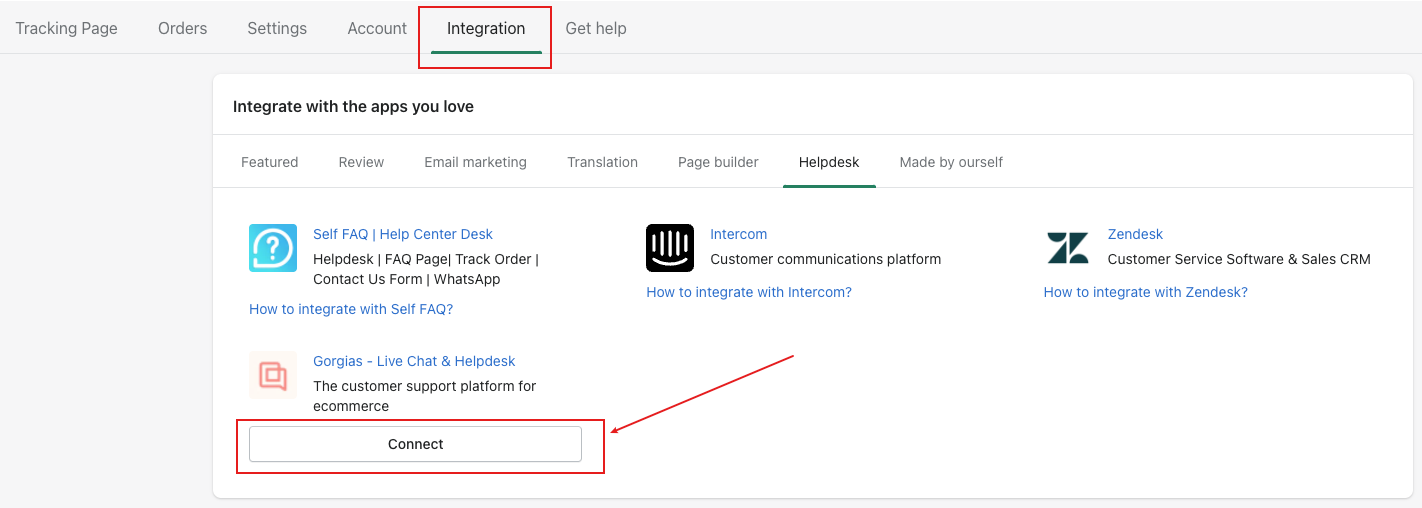The image depicts a user interface with a long horizontal navigation bar at the top. The bar includes tabs labeled "Tracking Page," "Order Settings," "Account," "Integration," and "Help." The "Integration" tab, situated fifth from the left, is highlighted by a green underline and a red border. Below this navigation bar, a white pop-up box appears, prominently displaying the text "Integrate with the apps you love" in bold black font.

The interface contains a section divided by lines above and below, detailing various features such as "Featured Review," "Email Marketing," "Translation," "Page Builder," "Helpdesk," and "Made by Ourselves." The "Helpdesk" feature is emphasized with bold text and another green underline.

Beneath the highlighted features, on the left side, there's a section labeled "Self FAQ Helpdesk," with clickable elements in blue, directing users to the help center. This section includes:
1. An image with a blue box featuring a white-bordered comment icon and question mark.
2. "Intercom," described as a customer communication platform, also featuring an image to the left.
3. "Zendesk," labeled as customer service software and sales, with hyperlinks on both "Zendesk" and "How to integrate."

The final highlighted feature in the "Self FAQ" section is "Gorgeous Live Chat Help," an e-commerce customer support tool. It includes a red box with a "Connect" button, marked by an arrow pointing upward to the right.